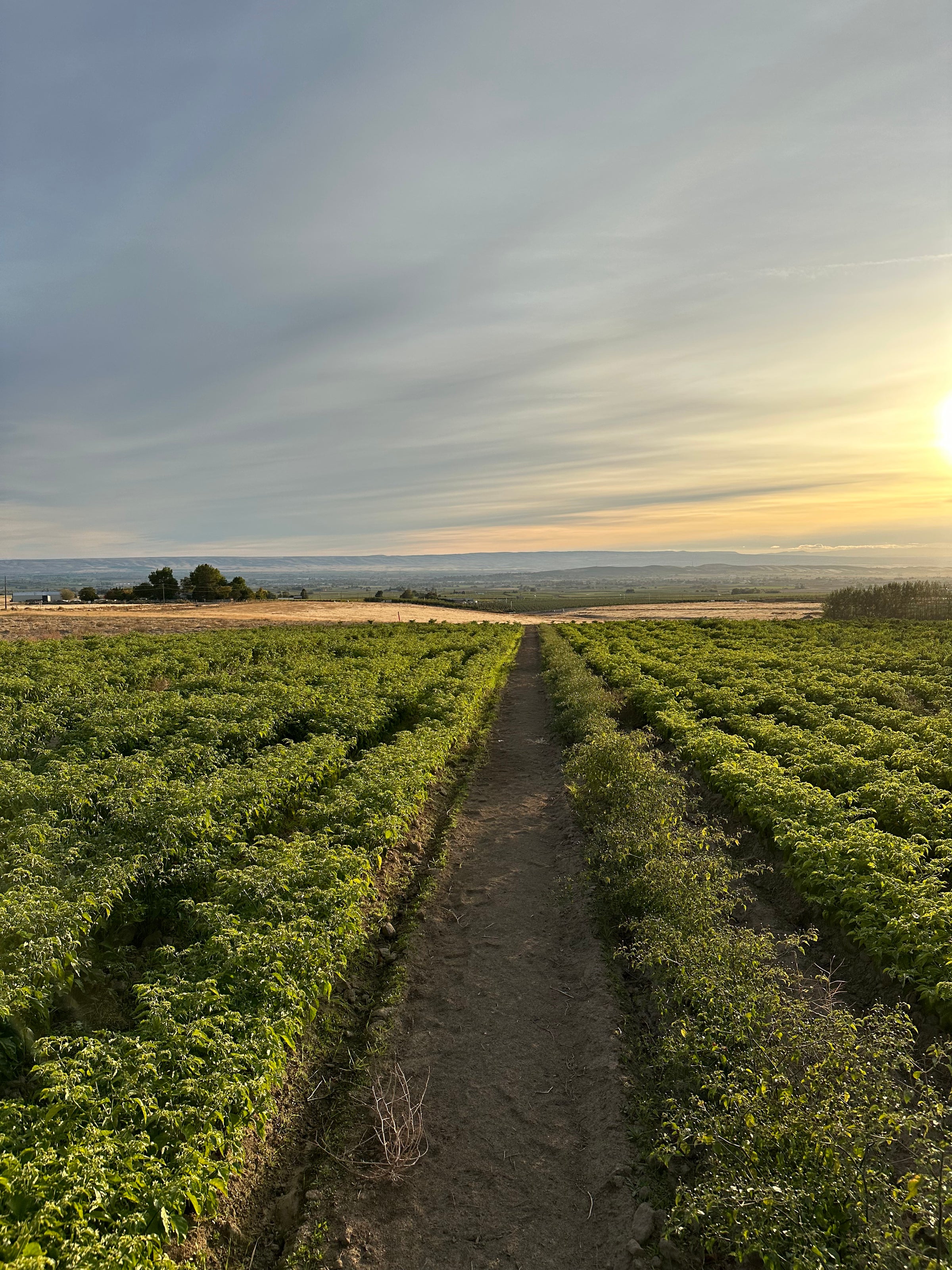The photograph captures a serene scene of farmland under an expansive sky. In the foreground, meticulously planted rows of what appears to be a leafy crop, possibly soybeans, stretch out in parallel lines. These green crops, resembling short bushes, are flanked by a brown dirt path or unplanted strip that runs from the bottom center to the distant horizon. The crops are vibrant and well-maintained, reflecting a healthy and weed-free growth. In the background, the color transitions to a sandy yellow, potentially indicative of a different crop like wheat, with dark green trees scattered across the landscape. Further back, faint mountain ranges add depth to the scene, while hazy elements suggest the presence of water. The sky above is mostly blue, interspersed with grayish-blue clouds. On the right side of the image, a bright yellow sun either rising or setting casts a golden hue across the sky, contributing to the tranquil beauty of the farmland.